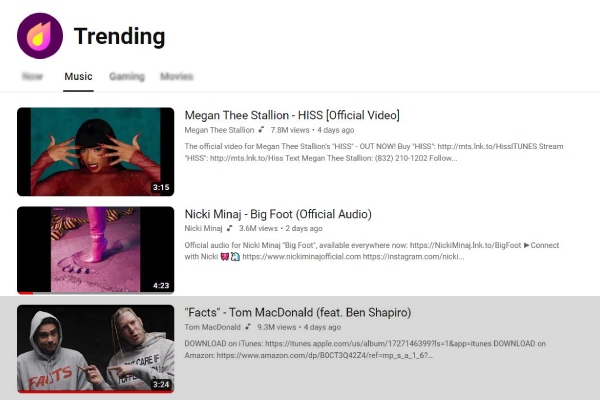On a white background, the top left corner features a dark purple circle with a purple and yellow flame icon in the center. To the right of this icon, the word "Trending" is displayed in bold black letters. Below this heading is a menu with four clickable options, among which the second option, labeled "Music," is highlighted while the others are blurred out.

Beneath the highlighted "Music" section are three YouTube video thumbnails. The first thumbnail at the top shows a woman with her palms facing her, positioned in front of her face, with the text "Megan Thee Stallion - HISS (Official Video)" overlayed. The second thumbnail, located below the first, displays a footprint in the sand, adjacent to a foot wearing high heels, accompanied by the text "Nicki Minaj - Big Foot (Official Audio)" to the right. The third and final thumbnail features two men in gray pullover hoodies with the caption "Facts - Tom McDonald featuring Ben Shapiro." The duration "3:24" is indicated at the bottom of this thumbnail.